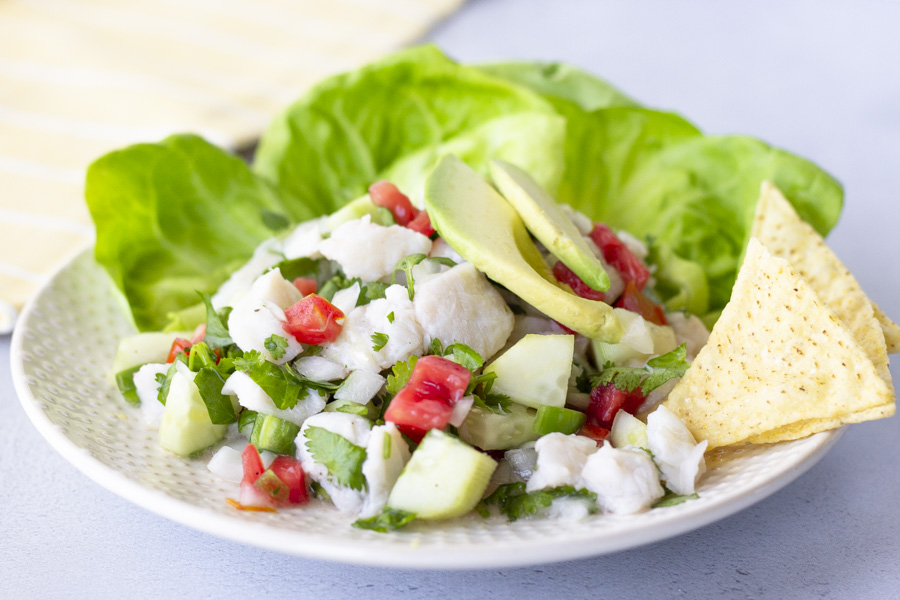The image showcases a vibrant and appetizing close-up of a salad served on a textured white plate with gently curved edges, giving it a shallow bowl-like appearance. Resting on a blue-gray background, possibly set on a napkin located in the upper left-hand corner, the plate holds a colorful assortment of fresh ingredients. Bright green lettuce leaves form the base, topped with lighter green sliced avocados, white chunks of what looks like cheese, and small red tomato cubes. Tucked into the right side of the salad are three or four rectangular tortilla chips in a light tan hue. The overall composition is sharp, clear, and bright, with sunlight or some form of direct lighting illuminating the dish from the left, resulting in a striking and mouthwatering visual.